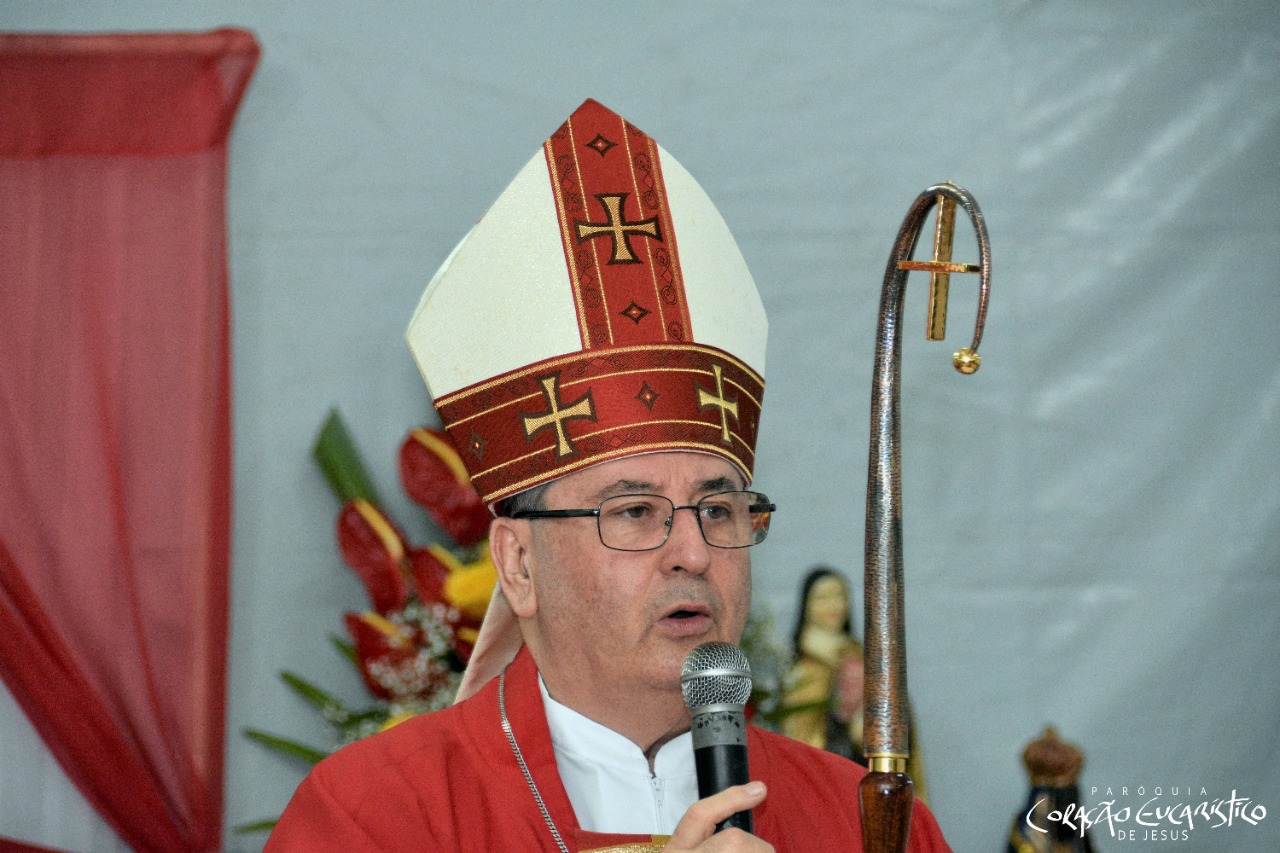The photograph features a distinguished bishop, an older gentleman with a stocky build and black-rimmed glasses, who is speaking into a black microphone with a silver top. He is adorned in ecclesiastical attire, wearing a red robe over a white tunic. Around his neck, he has a silver chain. His head is graced by a traditional miter, which is predominantly white with red striping adorned with gold crosses. He holds a scepter to his left; the scepter is wooden with a metal part culminating in a golden circle and cross at the top, resembling a shepherd's hook with a cross in the middle.

The background is slightly blurry, depicting floral arrangements, a statue of the Virgin Mary, and a red curtain to the left. The wall behind him is white, and there's another statue in the lower right of the image along with white lettering that reads "Caracciao Cucharistico of Jesus," indicative of the cathedral's name where this photograph was taken.